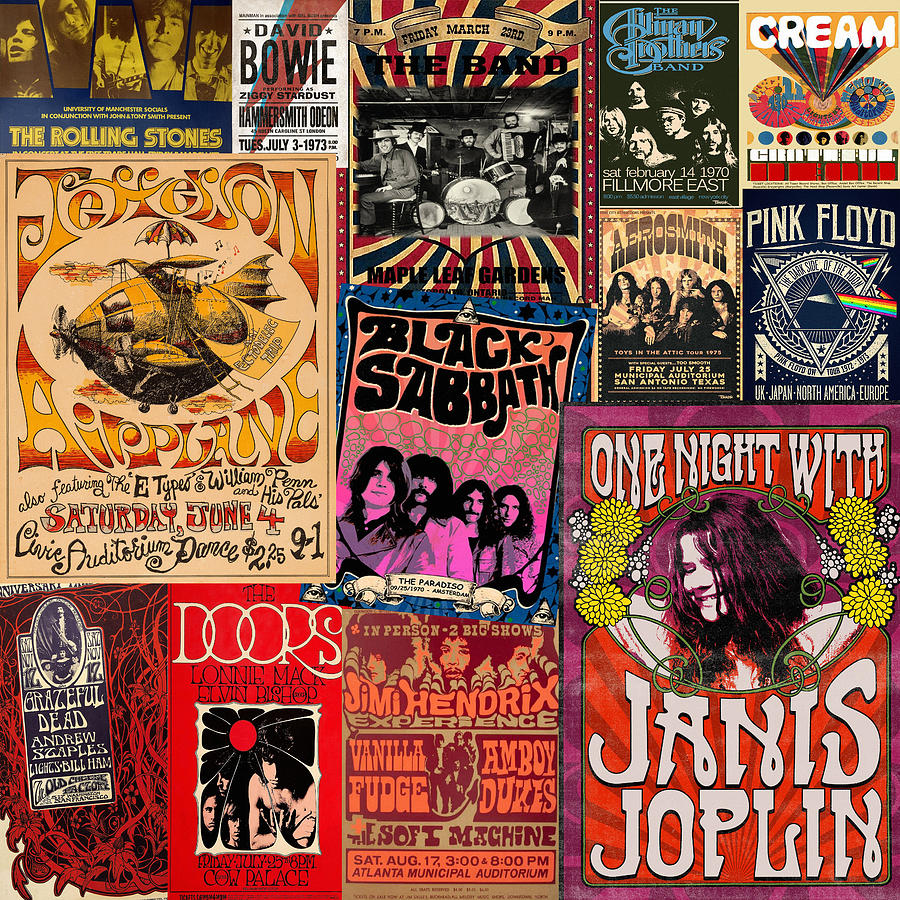This detailed composite image showcases a vibrant collection of vintage promotional posters for iconic musicians and bands from the 1950s to the 1980s. Dominating the top left, a Rolling Stones poster features a navy blue background with yellow and brown images of the band members. Adjacent to it is a striking David Bowie poster set against a white backdrop, adorned with a prominent red and blue lightning bolt and black lettering highlighting Ziggy Stardust. Next is a red, white, and blue Maple Leaf Gardens poster with a black-and-white photo of the band and clear white and black text.

Moving right, an eye-catching poster for Cream stands out with its cream-colored background accentuated by blue, yellow, red, and purple circles. Nearby, a Jefferson Airplane poster combines creamy hues with vibrant yellow and red text, featuring an iconic airplane illustration and red date lettering. The Black Sabbath poster captivates with its gradient background that shifts from blue to pink, adorned with black objects and white stars, complemented by a photo of the band outlined by bubble-like circles.

Beneath these, an Aerosmith poster displays a cream background with pink accents, presenting the band's name in bold black letters. The Pink Floyd poster is embellished with their signature symbols, including intertwined triangles and a rainbow motif, set against a stark white backdrop. Below this, a Grateful Dead poster swirls with red patterns against a dark background, while The Doors' poster pops with its bold red background and large white lettering.

In the lower section, a Janis Joplin poster catches the eye with a pink and red background, framed by yellow flowers and white bubbles, promoting "One Night with Janis Joplin." The Jimi Hendrix Experience poster stands out with orange lettering and a central image of Hendrix surrounded by unidentified figures, set against a layered white and dark brown background.

Each poster varies in style and color scheme but collectively conveys the dynamic and eclectic spirit of the music scene from this golden era.